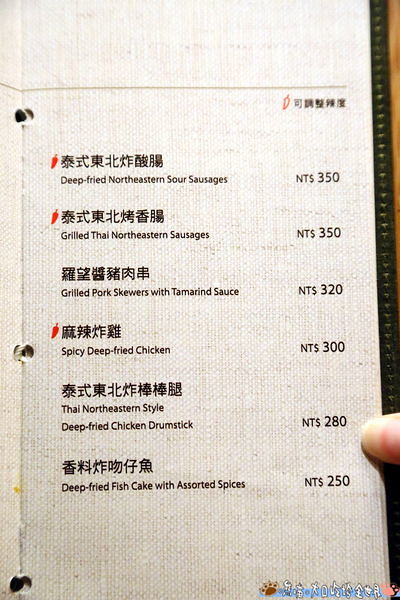The image captures the right-hand side of a rectangular menu booklet, taller than it is wide. The menu page has a light brown, woven fabric background, offering a rustic yet upscale quality. The page is bound by three punch holes with white string visible along the center crease. The edge of the menu is bordered in black, and at the bottom right, a Caucasian thumb is pressing against it. 

On the left-hand side of the page, each dish name is first presented in Chinese characters, followed by the English translation. A small red chili pepper icon indicates the spiciness of certain dishes. The list includes:

1. **Deep-Fried Northeastern Sour Sausages** - NT$ 350
2. **Grilled Thai Northeastern Sausages** - NT$ 350
3. **Grilled Pork Skewers with Tamarind Sauce** - NT$ 320
4. **Spicy Deep-Fried Chicken** - NT$ 300
5. **Thai Northeastern-Style Deep-Fried Chicken Drumstick** - NT$ 280
6. **Deep-Fried Fish Cake with Assorted Spices** - NT$ 250

The menu’s textured, muslin-like appearance, combined with its grainy brown detail and spaced-out text, captures a sense of both refinement and rustic charm.